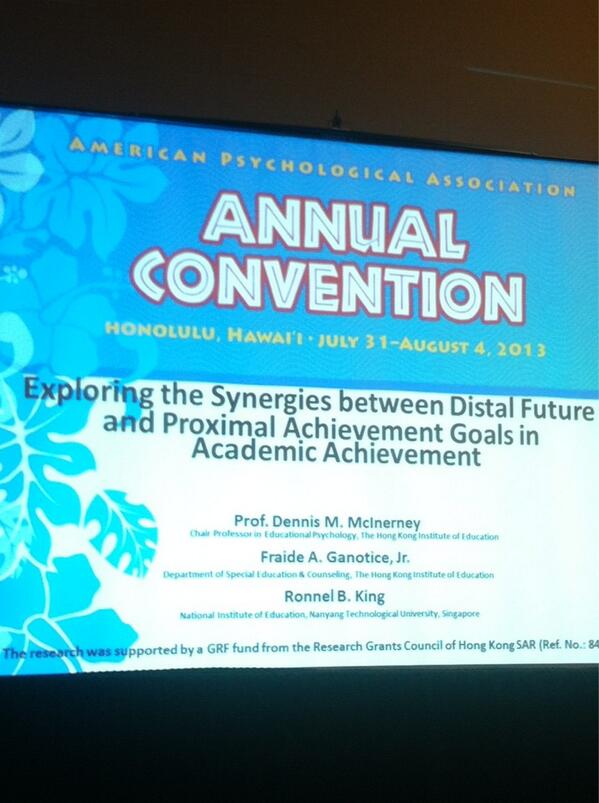This color photograph captures a screen projection, likely from a PowerPoint or conference presentation, set against a predominantly blue and white background. The top of the screen displays the text "American Psychological Association Annual Convention" in gold, followed by "Honolulu, Hawaii July 31st to August 4th, 2013." Below this, in large white letters, is the title of the presentation: "Exploring the Synergies Between Distal Future and Proximal Achievement Goals in Academic Achievement." The slide then lists the presenters: Professor Dennis M. McInerney from the Hong Kong Institute of Education, Fred A. Ganotis Jr. also from the Hong Kong Institute of Education's Department of Special Education and Counseling, and Ronell B. King from the National Institute of Education, Nanyang Technological University, Singapore. The lower part of the slide notes that the research was supported by a GRF fund from the Research Grants Council of Hong Kong SAR. The screen features a vibrant design with turquoise leaves and floral elements on the left side, evoking a Hawaiian theme.